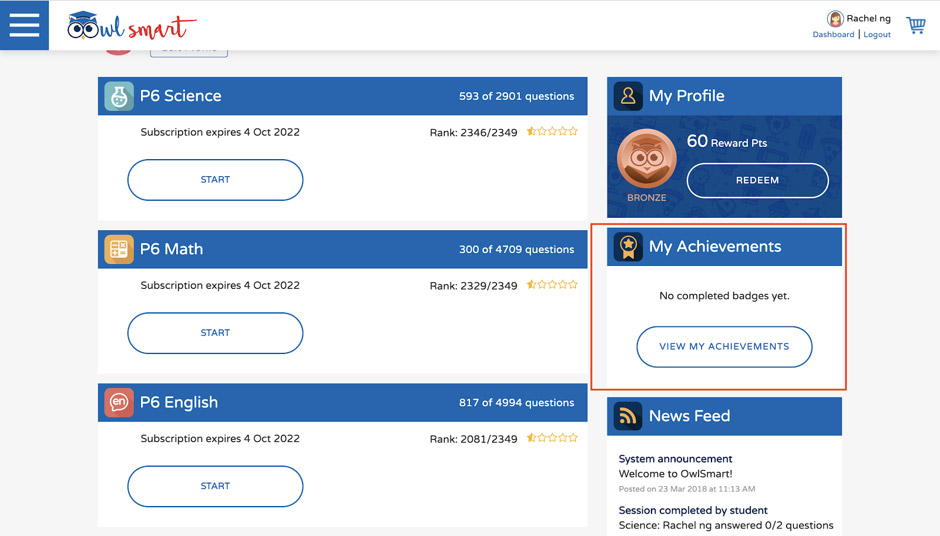In the upper left corner of the image, there is a blue square with three horizontal white lines stacked on top of each other. Adjacent to this, the text reads "Owl Smart" in a blue and red cursive font; the "O" is stylized as an owl face wearing a graduation cap. This text appears on a white strip. Toward the right, the text "Rachel NG" is displayed, and underneath it, there are buttons labeled "Dashboard" and "Logout" in blue font. On the far right, there's a blue shopping cart icon.

Below this section, the text reads "PG Science," indicating 593 of 2,901 questions completed. The subscription is stated to expire in October 2022, with a rank of 2,346 out of 2,349 and accompanied by a half-star rating. A white "Start" button with a blue outline and the word "Start" in blue text is situated below this.

Further down, another section has a blue strip at the top, indicating a similar format. This one refers to "PG AP6," with 300 of 400,709 questions completed. The subscription also expires in October 2022 with a ranking of 2,032 out of 2,349, also with a half-star rating. Below this is another white "Start" button outlined in blue, with the word "Start" in blue text.